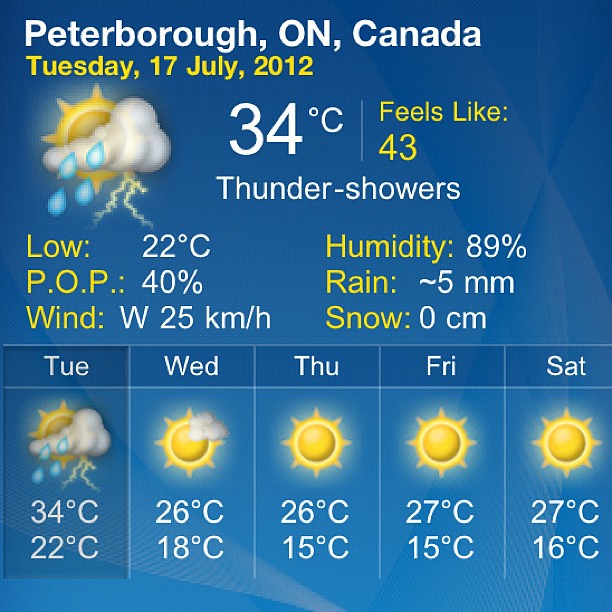The image is a digitally displayed weather report for Peterborough, Ontario, Canada, set against a deep blue patterned background. In the top left corner, in bold white font, it reads "Peterborough, ON, Canada," and below that, in bright yellow font, "Tuesday, 17 July 2012." Adjacent to this text is an icon depicting a sun partially obscured by a puffy white cloud, with four blue raindrops and a yellow lightning bolt emanating from it. Directly to the right, the temperature reads "34 degrees Celsius," and below that, in yellow, "feels like 43." Beneath this information, in white font, it states "Thundershowers." Additional weather data follows, noting a low of "22 degrees Celsius," "Humidity 89%," "POP 40%," "Wind W 25 km/h," "Rain 5 mm," and "Snow 0 cm." At the bottom of the image, a five-day forecast chart displays icons of a sun with varying conditions from "Tuesday" through "Saturday," with associated weather conditions and temperatures listed beneath each day.